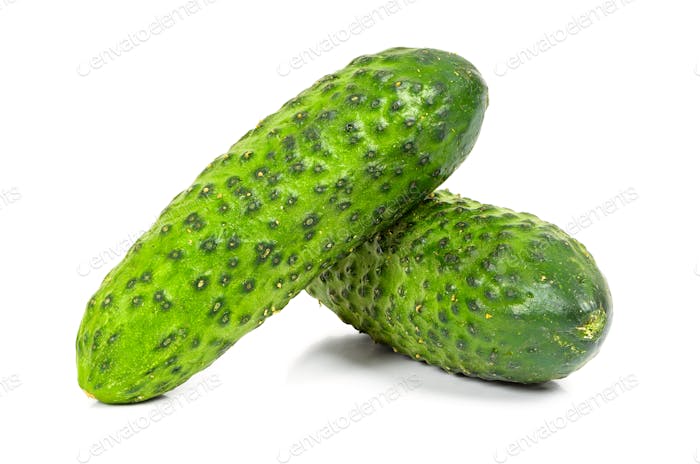The image features two cucumbers or pickles, vividly displayed against an all-white background. The cucumber on top leans at an angle over the one lying flat below. Both vegetables are characterized by a notably bumpy texture with dark spots resembling black zits, varying in shades from medium to light green. The upper cucumber appears lighter with distinct shadowing that emphasizes its contours. There is a faint and difficult-to-read brand watermark, suggesting "Senvato Elements," adding a possible promotional or artistic context. The background and composition imply that these might be fresh cucumbers that are yet to be pickled, highlighted in what could be an online grocery advertisement or a professional food photograph.